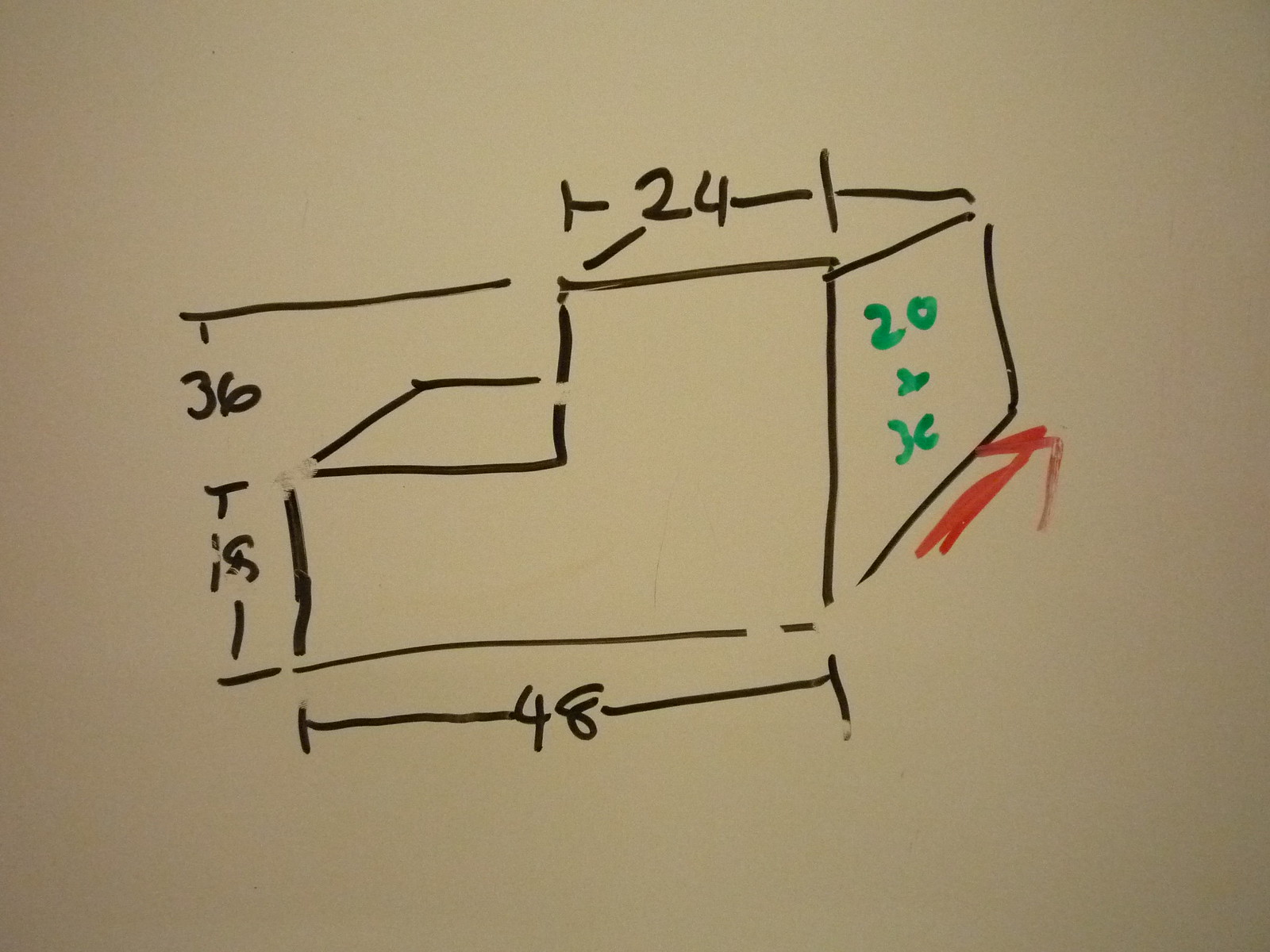The image depicts a hand-drawn schematic of a two-step structure, featuring detailed measurements in various colors of markers. The first step is labeled with a width of 24 units, while the second step has a width of 36 units. The combined height of the two steps is denoted as 48 units. There is a dimension line extending from the front to the back of the drawing, marked clearly with "48". Additionally, the width of the steps is highlighted in yellow, with a red arrow spanning side to side. There is also a green pen notation that reads either "20 and 36" or "20 and 30" (the latter part being somewhat illegible, possibly resembling "3C"). Most of the measurements are written in black or dark purple marker, making them easier to read compared to the green notations.